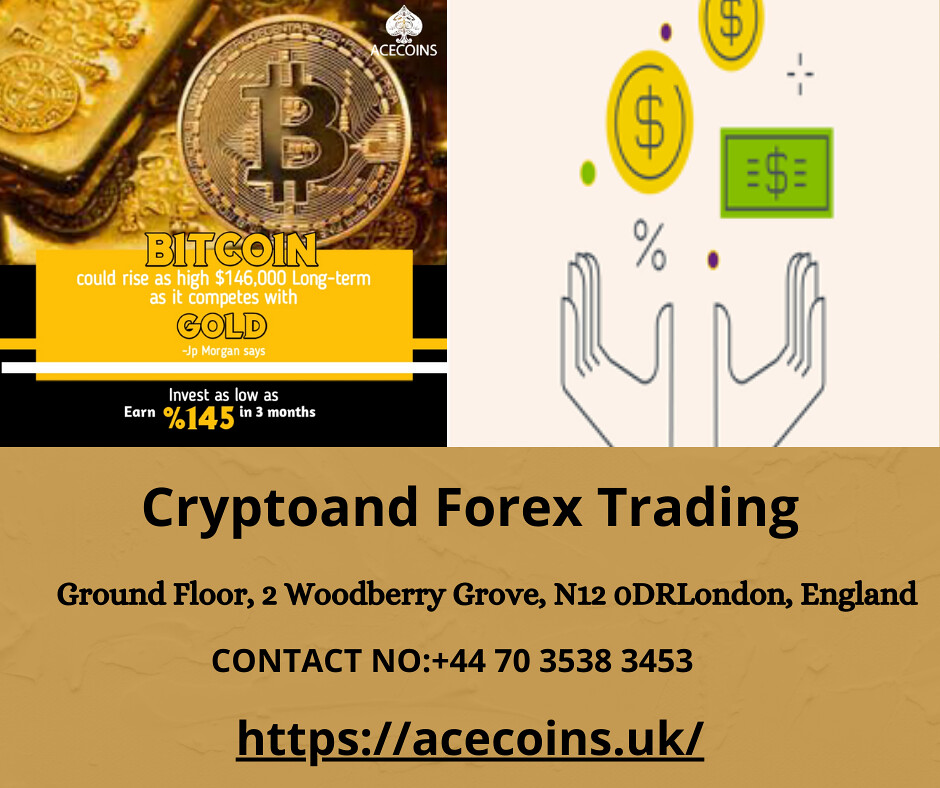This online advertisement is visually divided into three sections. The top left section features a golden Bitcoin coin juxtaposed with gold bars. Accompanying this imagery, a prominent yellow caption states, "Bitcoin could rise as high as $146,000 long-term as it competes with gold," quoting JP Morgan. It also mentions investment returns of up to 145% in three months. On the right side, there's a graphic illustration of hands raised upwards, with gold coins and dollar bills falling down, symbolizing wealth and financial gain. The bottom portion has a brown background with black text providing business details: "Crypto and Forex Trading," located on the ground floor at 12 Woodbury Grove, N12 ODR, London, England. Contact information includes the phone number +44 703 538 3453, and the website https://acecoins.uk. The entire setup aims to encourage investment in cryptocurrencies and forex trading.